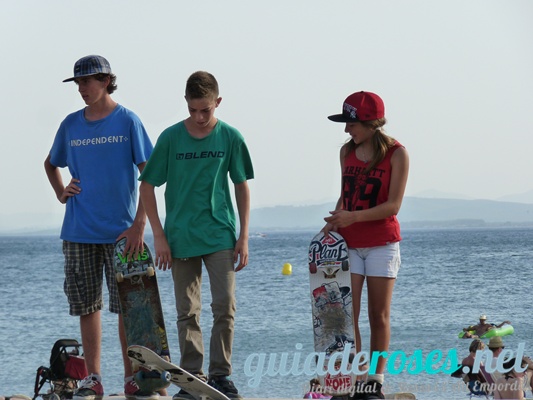A photograph captures three young teenagers standing in front of a vast body of water, possibly an ocean, with distant mountains and people enjoying the waves on inflatable tubes. The trio appears to be on a firm surface with some skateboarding equipment scattered below, suggesting they are not on sand. The young man on the left sports a blue T-shirt with "Independent" written in white, checkered shorts, and a baseball cap. He holds a skateboard upright beside him. The boy in the center, dressed in a green T-shirt with khaki pants, gazes downward while standing on one end of his skateboard, causing the opposite end to lift. On the right, a girl wearing a red tank top with black lettering, white shorts, and a red cap with a dark bill holds her skateboard. Her top displays the number 89. The sky above is bright, indicating a clear day with a gentle wind. None of the three adolescents are looking directly at the camera, making the moment feel candid and spontaneous.